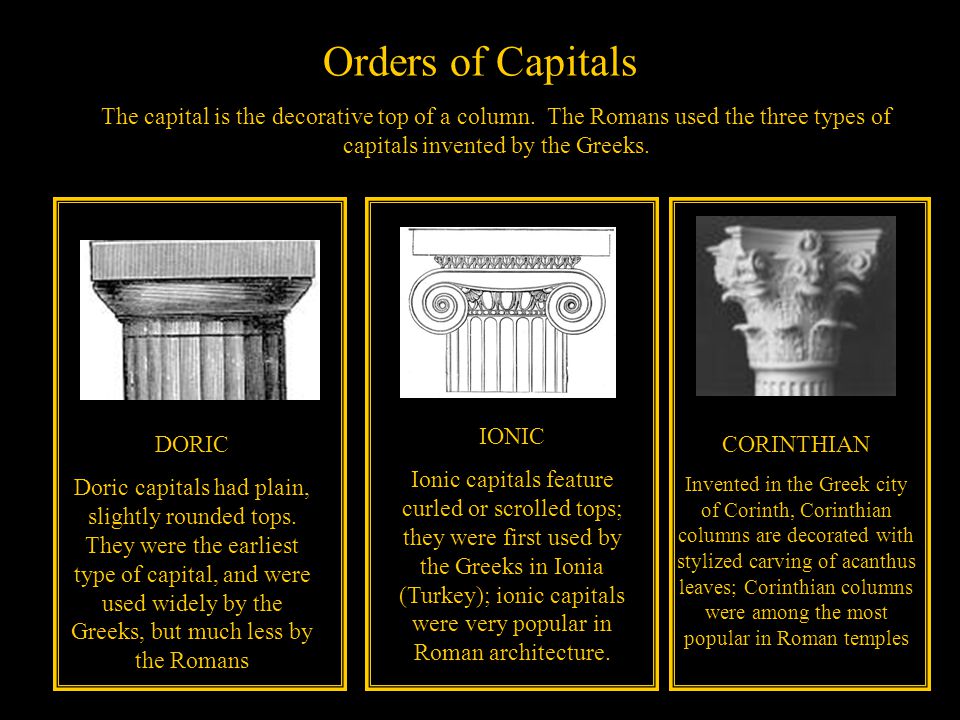The image is a detailed slideshow titled "Orders of Capitals" in orange letters against a black background. It features ornate illustrations and descriptions of three types of column capitals used by the Romans, originally invented by the Greeks. On the left, the Doric capital is depicted with its plain, slightly rounded tops. These were the earliest type and were widely utilized by the Greeks, but much less so by the Romans. The middle column shows the Ionic capital, distinguished by its curled or scrolled tops, first used by the Greeks in Ionia, Turkey, and very popular in Roman architecture. On the right, the Corinthian capital is illustrated, noted for its elaborate carvings of acanthus leaves, and it was among the most favored designs in Roman temples. Each column has corresponding yellow text explaining its origins and characteristics, providing a comprehensive overview of these architectural elements.